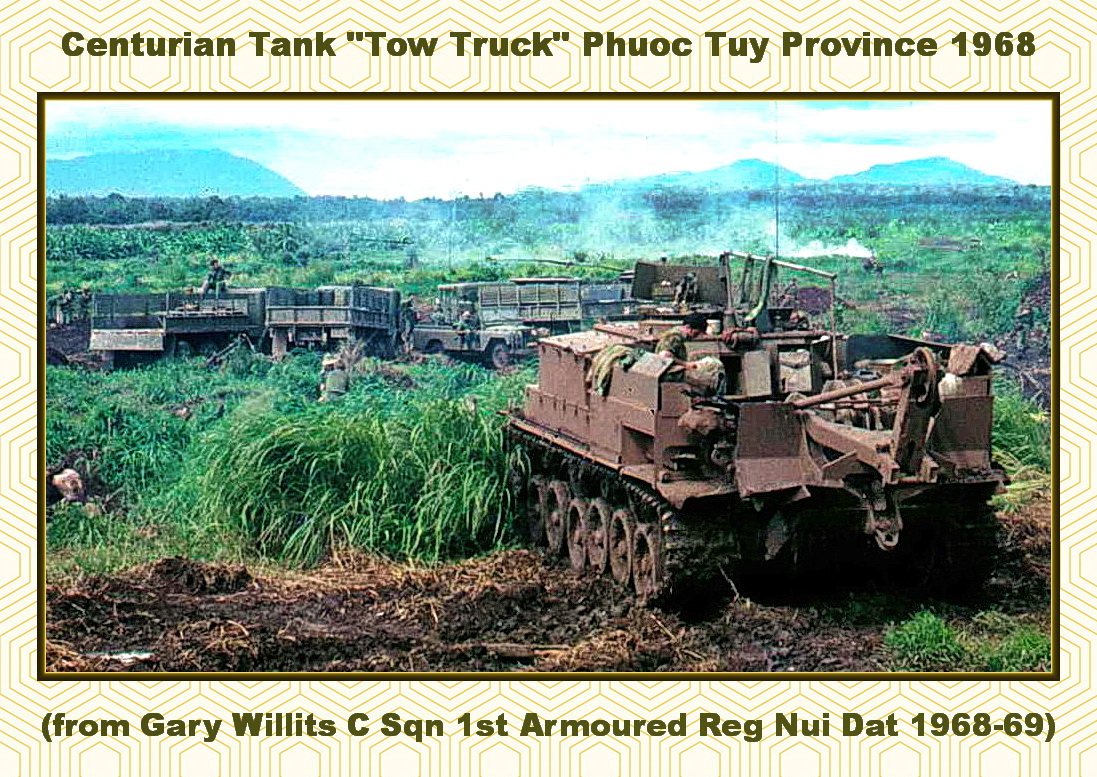The image resembles a vintage postcard featuring a centrally placed photograph outlined by a black frame and surrounded by a white background with a subtle pattern. At the top of the card, in dark green or black lettering, it reads: "Centurion Tank 'Tow Truck', Phuoc Thuy Province, 1968." At the bottom, in parentheses, it states: "From Gary Willett's C SQN, First Armored Reg, Nui Dat, 1968-69." 

The photograph itself is a historical scene capturing a grassy, muddy field with various military elements. In the lower right corner, there is a Centurion tank, dark brown and green, equipped with tracks and a turret, with a person visible on the back. Facing away from the viewer and slightly to the left, the tank sits near some tall grass. To the left side of the image, there are several army trucks, a jeep, and soldiers either seated or atop the vehicles. Smoke rises in the distance, creating an atmospheric backdrop against the distant hills and an overcast sky.